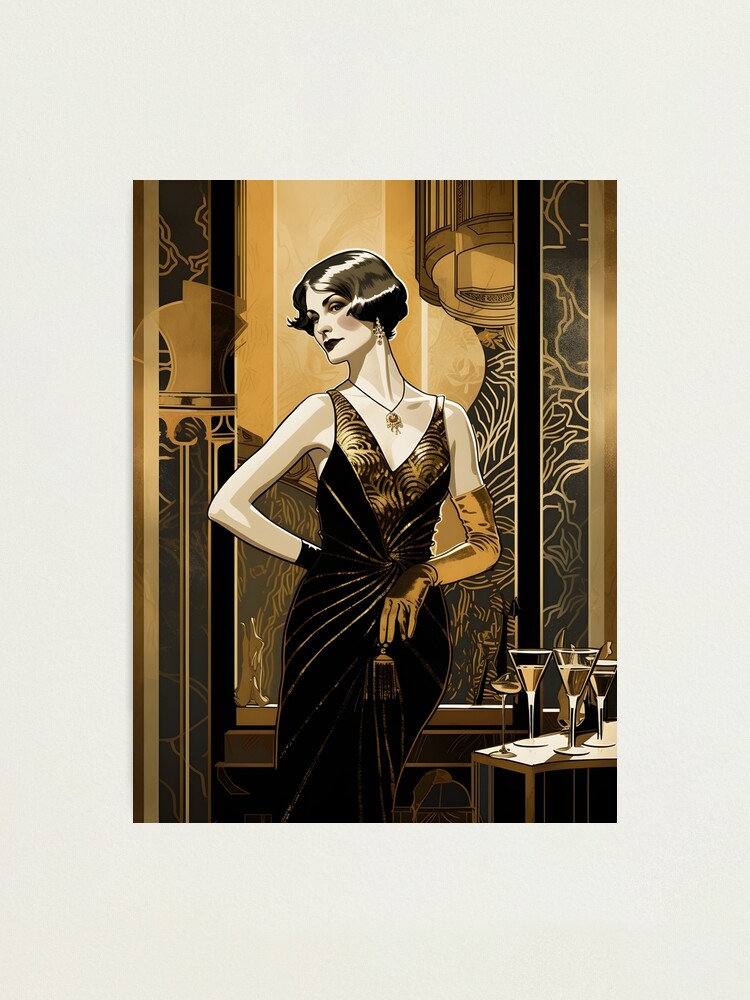This promotional image, designed to sell a high-quality poster, painting, or canvas print, features an elegant drawing of a woman from her knees upward. Set against a digitally edited white background that mimics a wall, the artwork emphasizes the luxurious use of gold and white, with subtle black accents. The woman is portrayed in a sleeveless, thin-strapped evening gown with a pronounced low V neckline, elegantly cinched at the waist to highlight her figure. She wears a long gold glove that extends above her left elbow and a contrasting black glove on her right hand, which rests on her hip. Her accessories include a black necklace adorned with a gold pendant, and dangling gold earrings, adding to her sophisticated appearance. The scene evokes a sense of early 20th-century glamour, reminiscent of the Gatsby era. Although there are references to alcoholic glasses and an intricate, metallic silver-gold backdrop, these elements are absent, suggesting the primary focus remains on the woman's timeless elegance.